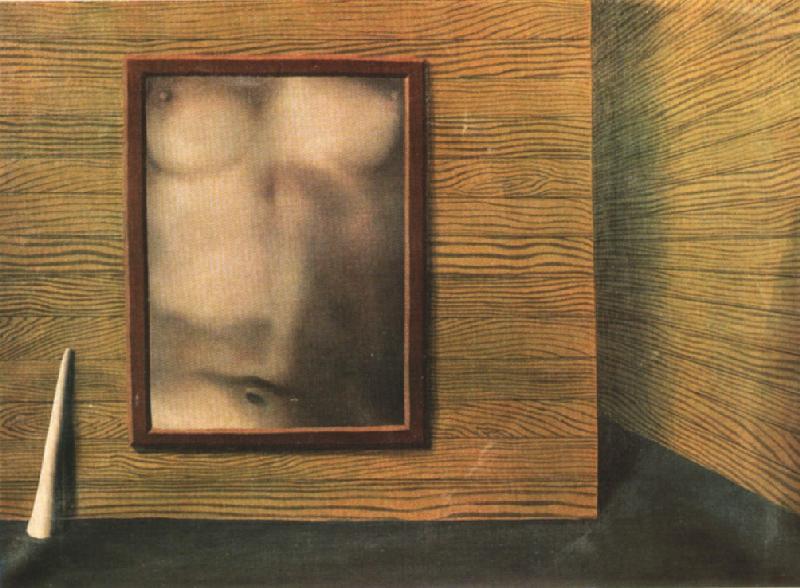The image portrays an unusual scene of a wooden-paneled room with horizontal planks lining the walls. The main wall features a brown-framed artwork that showcases a nude torso, depicted in a contrasting style to the room's rustic aesthetic. The torso, with defined pectorals, a flat abdomen, and a visible navel, presents some ambiguity regarding its gender, as it shares characteristics of both male and female forms. Adjacent to the wooden wall, a peculiar, long, pointed object resembling an oversized golf tee leans nonchalantly, adding an element of mystery. The floor beneath is a solid, dark gray surface, possibly painted concrete, adding to the room's minimalist yet compelling composition.